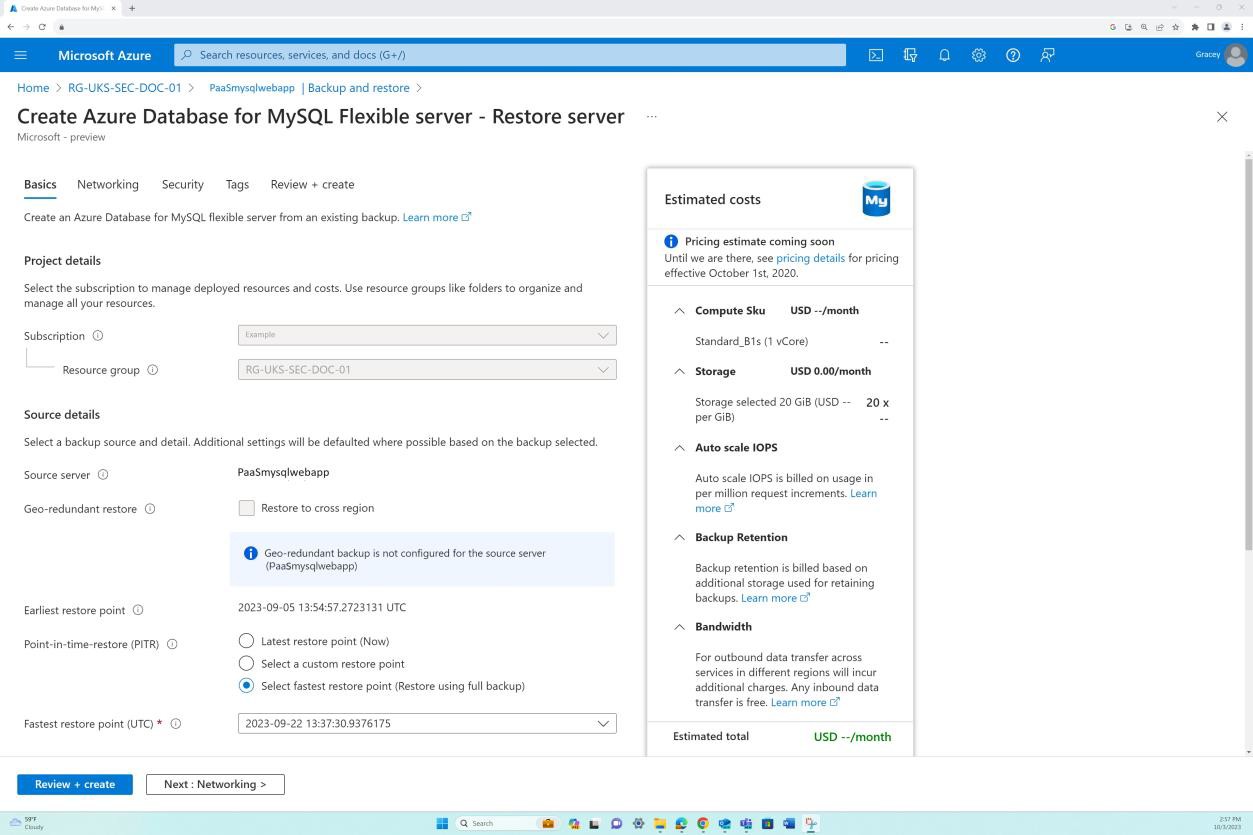The image depicted is a screenshot from the Microsoft Azure website, clearly highlighting various interface elements. The top section of the screenshot displays a series of narrow gray rectangles, which are input fields designed for navigating to different tabs within the Azure portal. Below this, a royal blue horizontal line prominently features the text "Microsoft Azure".

Immediately beneath this line is a search bar labeled "Search resources, services, and docs," facilitating user queries within the Azure ecosystem. As the image progresses downward, a notable section is dedicated to creating an Azure Database for MySQL Flexible Server, specifically for restoring a server from an existing backup. This section includes various configurable settings denoted by tabs such as "Basics," "Networking," "Security," "Tags," and "Review + create".

To the right side of this section, the image displays an area outlining the estimated costs associated with the service, with specific estimations effective from October 1, 2020. Further down, on the bottom left of the image, are two crucial buttons: a blue "Review + create" button and a "Next: Networking" button. These elements guide the user through the process of configuring and deploying their Azure Database for MySQL Flexible Server.